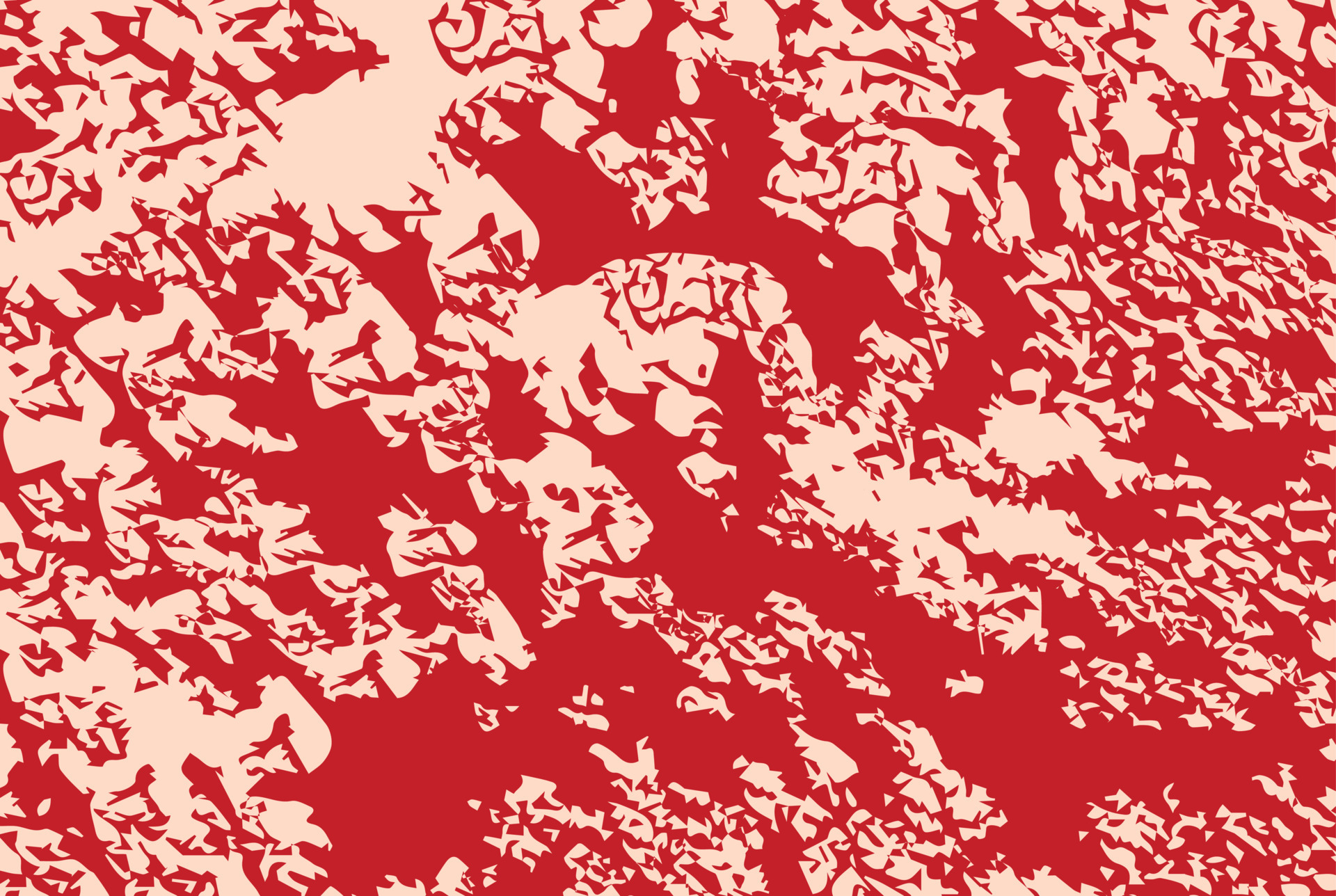The image is a large rectangular poster featuring a dynamic and busy abstract painting. The primary colors are a salmon pink and a deep red, creating a visually striking contrast. The background appears to be painted pink, with red paint applied on top, which has been intentionally chipped or wiped away in various areas. This random and unstructured removal of the red paint reveals intricate shapes and patterns that intermingle, forming a variety of interpretations. Among the angular and sometimes jagged lines, viewers can discern shapes that resemble dogs, sharks, and even human faces, although these forms are not uniform and lack a clear focal point. On the left side of the poster, larger shapes dominate, gradually transitioning into smaller shapes towards the right, offering an intriguing play of size and density. The overall effect is a non-uniform, multi-faceted design that captivates the observer with its complexity and the interplay between the pink and red hues.